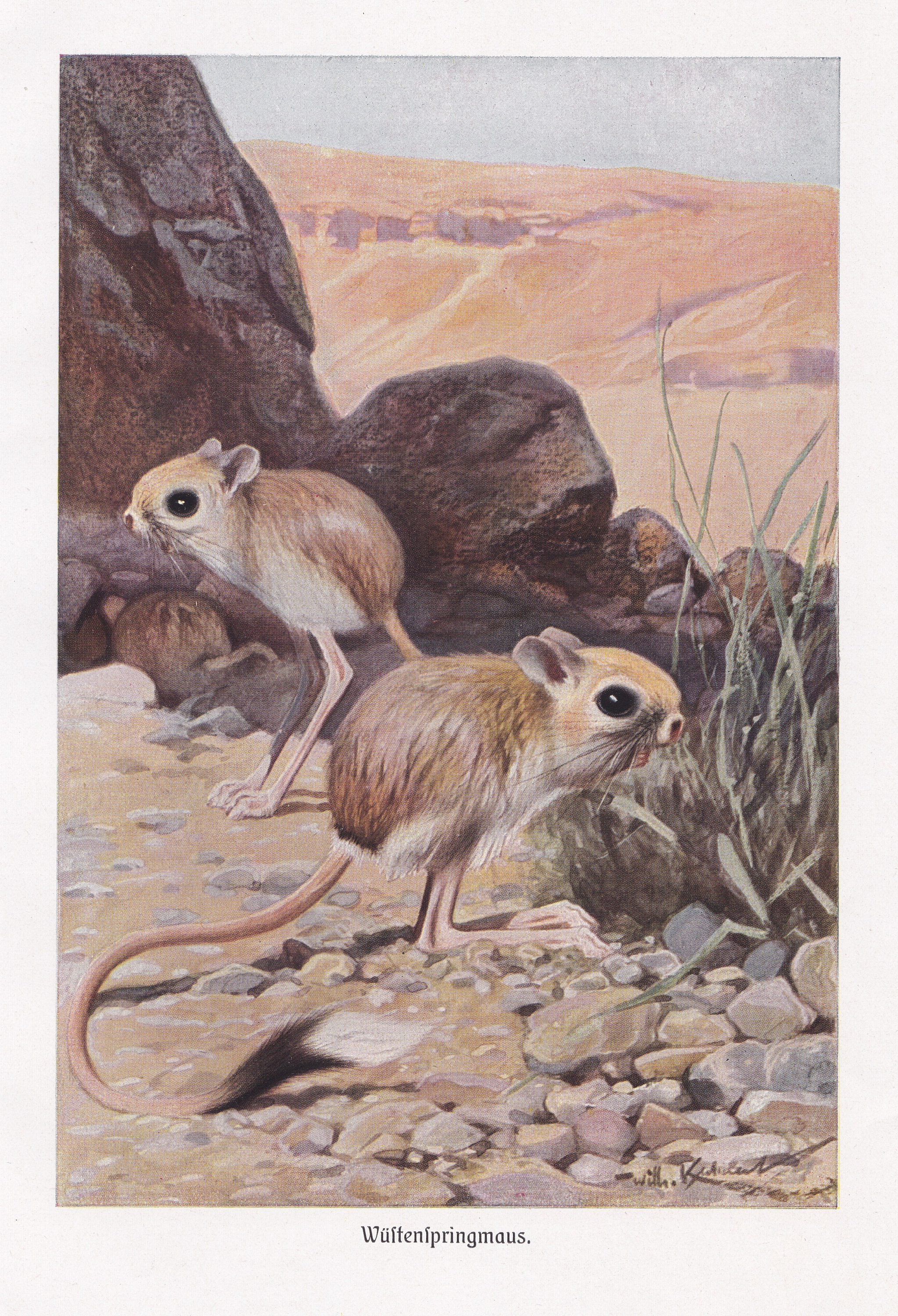This image is a color illustration on a white border featuring a desert scene with peculiar mouse-like creatures. The illustration depicts three small brown animals with distinct characteristics: they have short, rounded ears, large black eyes, and long, kangaroo-like legs. Their bodies are round and furry, extending into long, hairless tails. In the foreground, one creature is crouched down facing right, while another stands tall on its hind legs facing left. A third one is in the distance, its back turned, investigating the rocky terrain.

The setting is a sandy, beige desert with gravel scattered on the ground. In front of the crouching creature, some grasses are visible. Dark grey rock formations rise behind the standing creature, leading into a vast desert landscape under a clear blue sky. At the bottom of the image, written in ornate text that appears to be German, is the phrase "Wältenspringmaus," indicating these are likely a specific type of spring mouse.